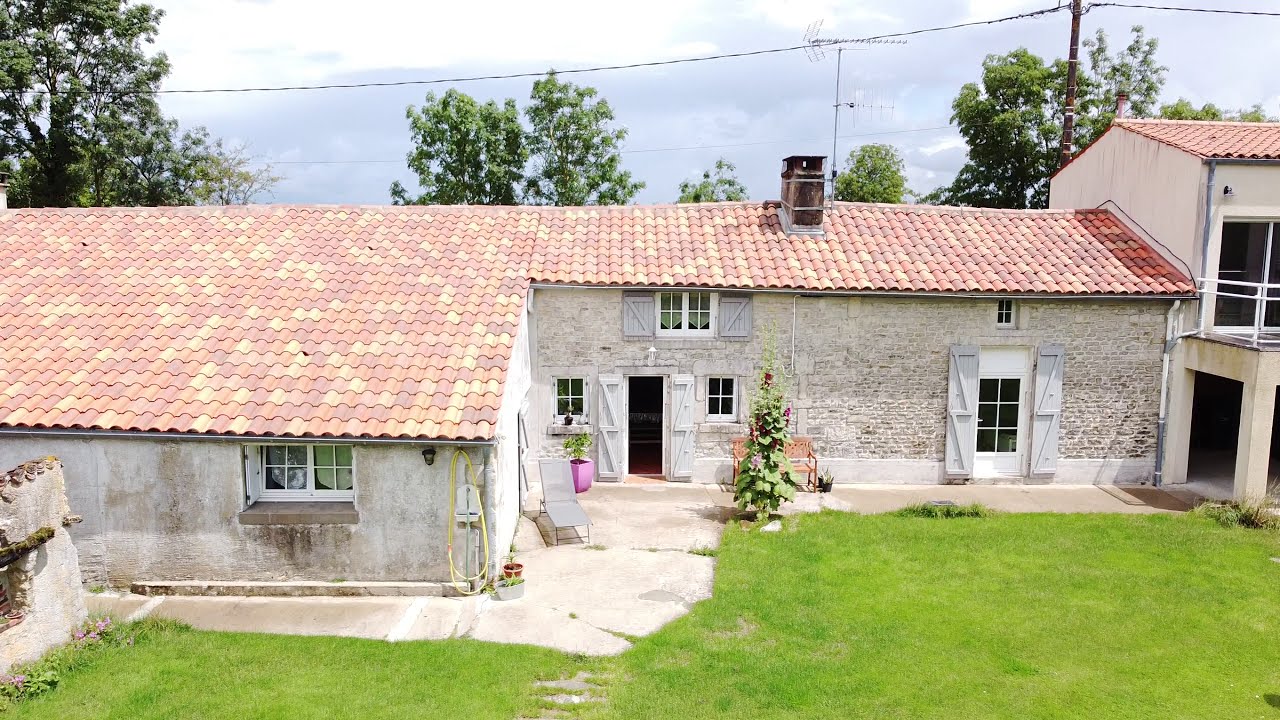The image depicts a historical-looking house, reminiscent of Mediterranean architecture commonly found in Portugal or Spain. The house has a distinctive red shingled roof composed of barrel-shaped clay tiles in varying shades of reds, oranges, yellows, and pinks. The structure is primarily gray, with some sections made of stone or brick and others appearing to be concrete. The elevation changes as it extends forward on the left side. The main entrance, which faces the camera, features white-trimmed windows with gray shutters on either side and wooden doors.

In front of the house, there is a small concrete sidewalk and a lush, green grassy lawn closer to the camera. The front area includes a concrete patio with a gray lounge chair and a brown bench, accompanied by three potted plants, adding to the picturesque scene. The right-hand side of the house is a two-level section, contrasting with the predominantly one-level structure. The bright, cloudy sky overhead reveals a backdrop of trees and utility wires, completing the quaint yet somewhat weathered look of this old, charming home.